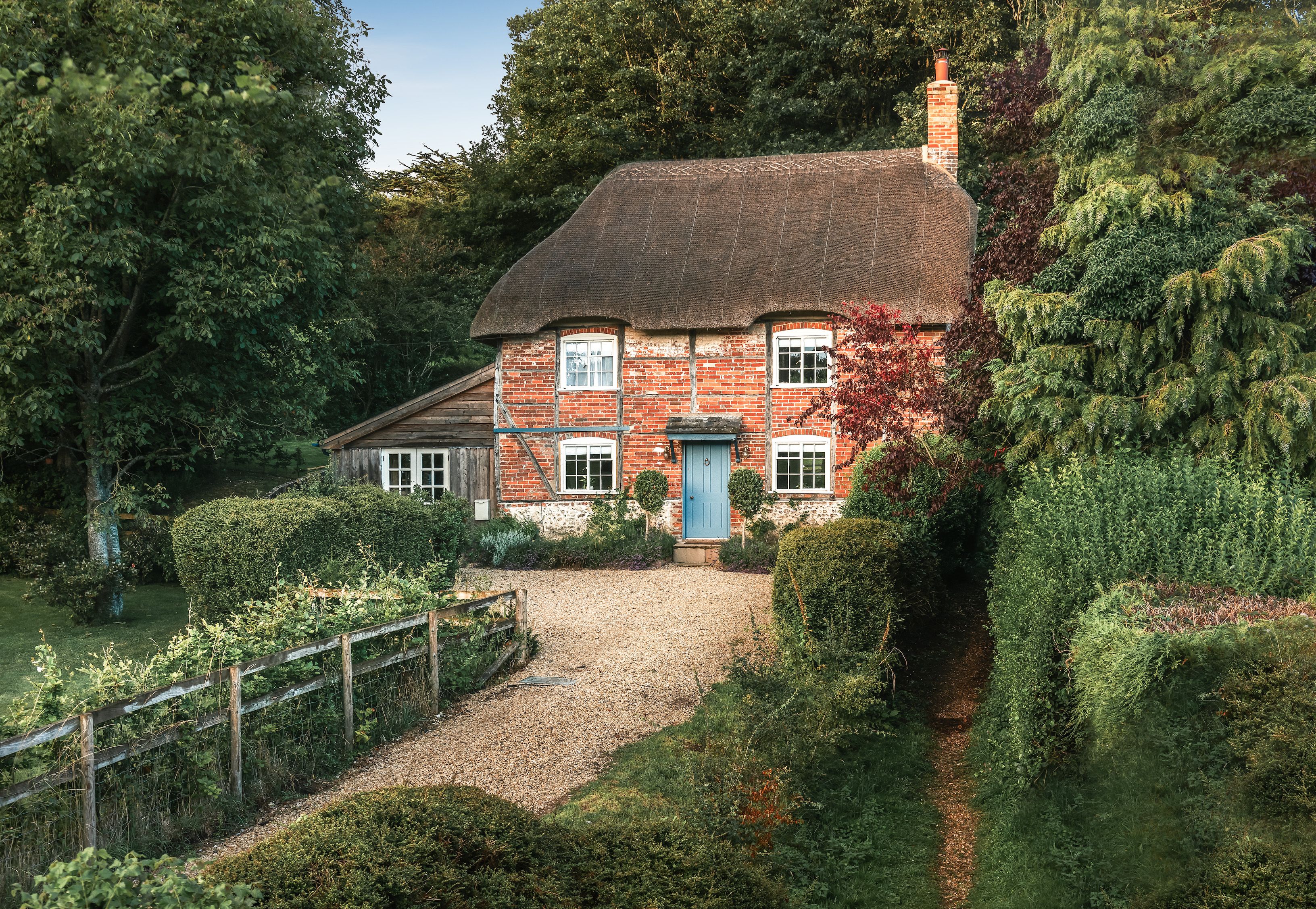This image captures an old, likely 19th-century, two-story cottage nestled in a lush forest setting. The cottage features an orange brick exterior and a very dark, perhaps mildewed, steeply sloped roof. The roof also has a red chimney poking out. Prominently displayed in the center of the home is a vibrant light blue door flanked by four white windows—two on the top floor and two on the bottom. Attached to the left side of the house is a wooden storage building or shop, which also has windows.

The house is framed by an abundance of green trees and well-manicured hedges, enhancing its sequestered feel. To the left of the property, there is a large tree and a small wooden fence, while a brown gravel driveway and pathway lead from the bottom left corner of the image up to the front door. A smaller red pathway can be seen trailing off on the right side among the hedges. The entire scene is bathed in sunlight under a clear blue sky, highlighting the serenity and idyllic nature of this secluded woodland cottage.